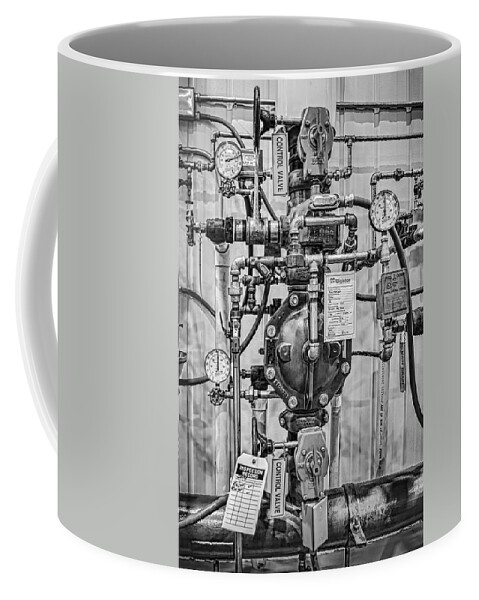This is a detailed photo of a white coffee mug featuring a complex black and white design. The design on the mug depicts an intricate assembly of various types of pipes, valves, and dials, resembling a water pump or similar mechanical fixture. Among the detailed elements, there are several paper tags affixed to different parts of the depicted machinery, including a legible tag that reads "control valve." The image on the mug is rich with detailed instrumentation and machinery, offering a monochromatic industrial aesthetic. The only hint that it is indeed a coffee mug is the barely visible handle towards the rear of the image.